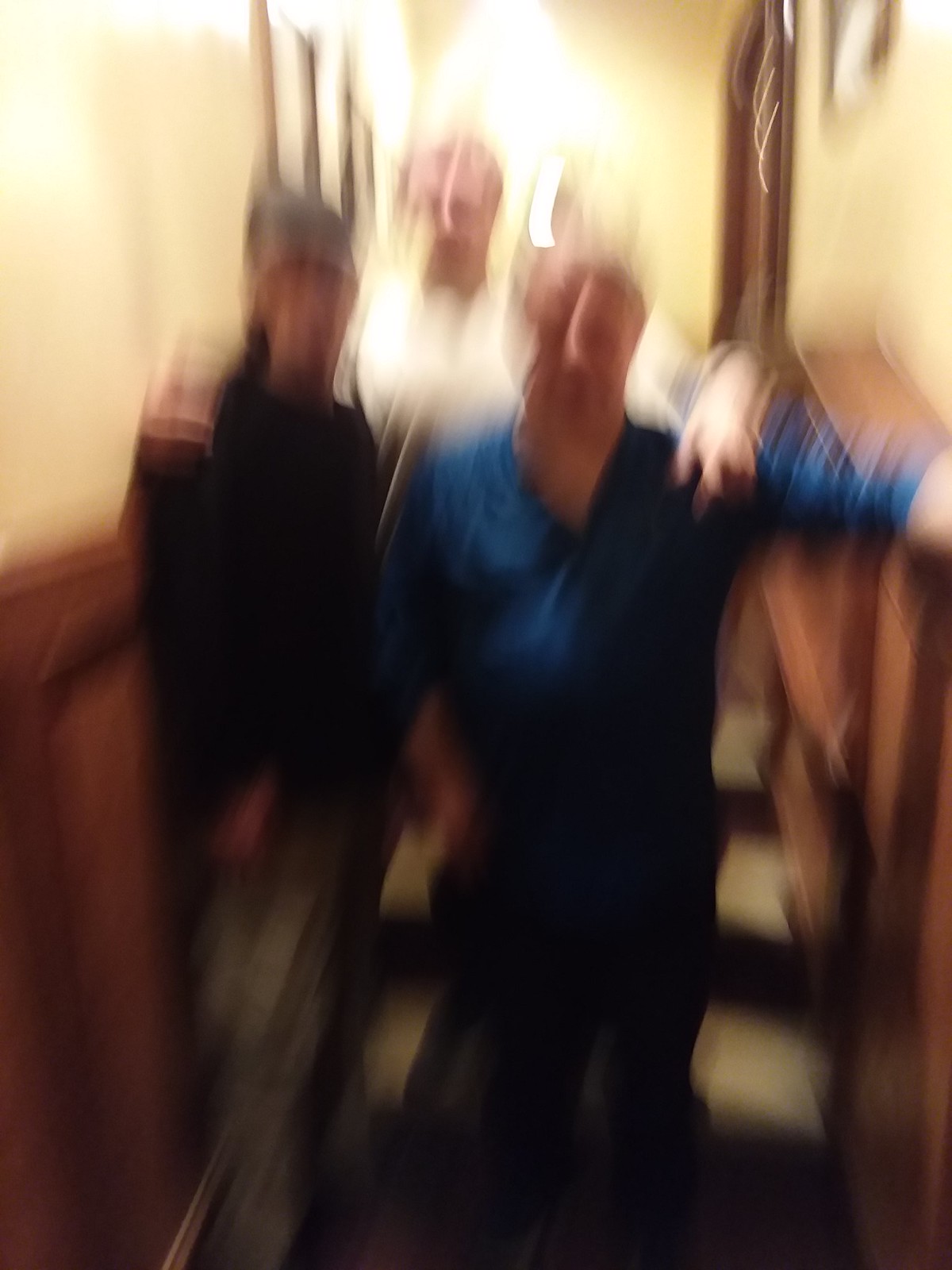In this blurry photograph, three men are posing in a narrow, dimly-lit hallway. Two men stand in the front, while a third man is positioned behind them, with his arms draped over their shoulders in a friendly gesture. All three men appear to be of a light-skinned, white ethnic background. 

The man on the front right is dressed in a blue long-sleeved shirt, which is rolled up to his elbows, and dark pants. Next to him, on the left, is a man wearing a dark shirt, gray pants, and a gray hat. The man in the back is sporting a white shirt, but his lower body is not visible in the frame. 

The hallway itself features wood paneling at the bottom, transitioning to a lighter color on the upper part of the walls. A spotlight behind the trio illuminates the scene, casting light on the wooden surfaces and adding a warm glow to the photograph, despite its blurry quality.